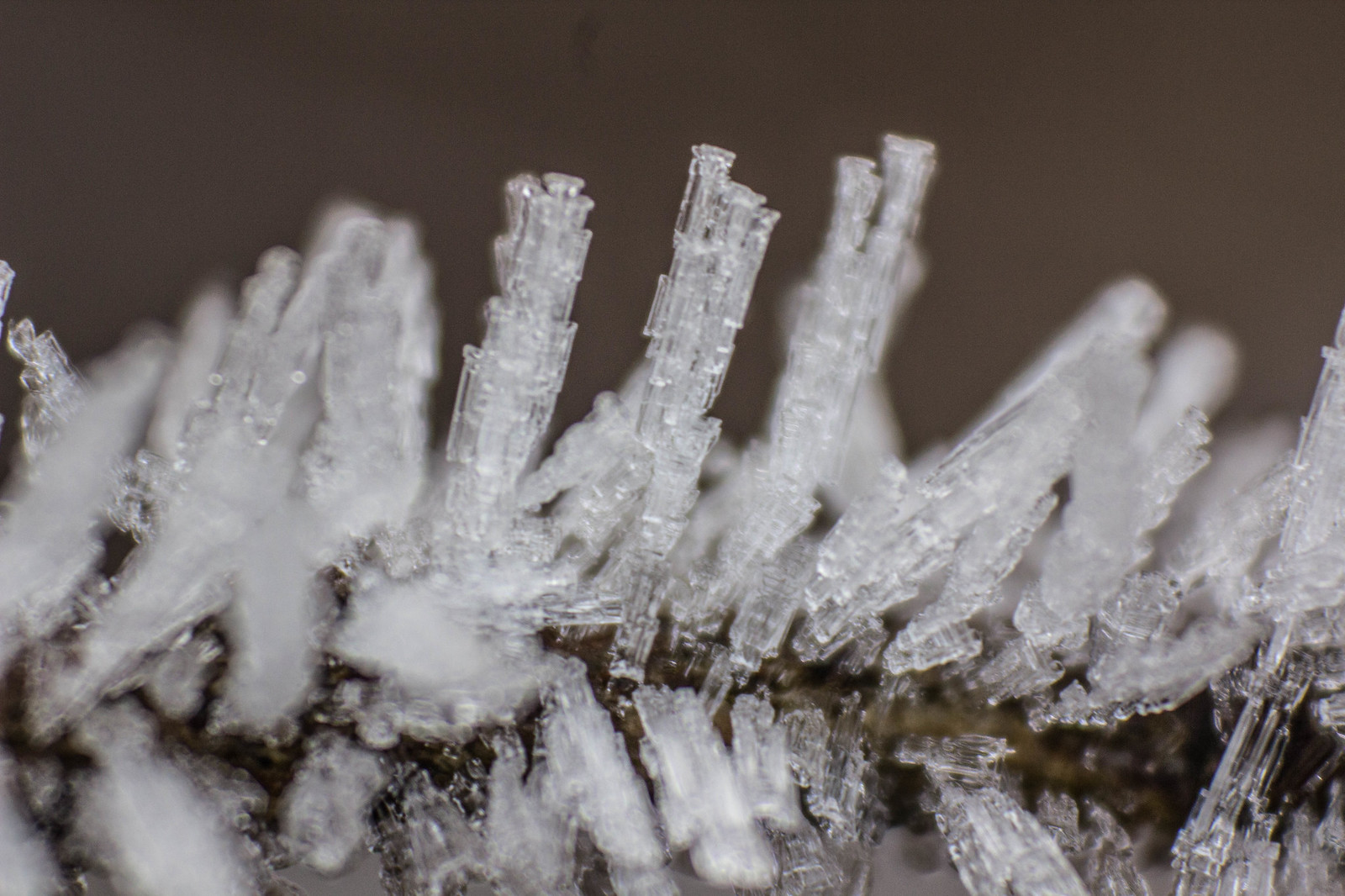This close-up photograph captures an intricate formation of ice crystals against a predominantly dark background. The ice crystals, which appear to be delicately adhering to a branch or a similar object, are arranged in various directions - sticking straight up, out, and sideways. The crystals exhibit a range of white, clear, and light-brown hues, giving them a glass-like appearance. These ice formations are composed of numerous segmented parts, some of which are cylindrical with flat tops. The background, mostly black with some dark brown and grayish tones, creates a stark contrast that highlights the delicate, crystalline structure. The image is notably magnified, allowing for detailed observation of the ice crystals' intricate patterns and segments.